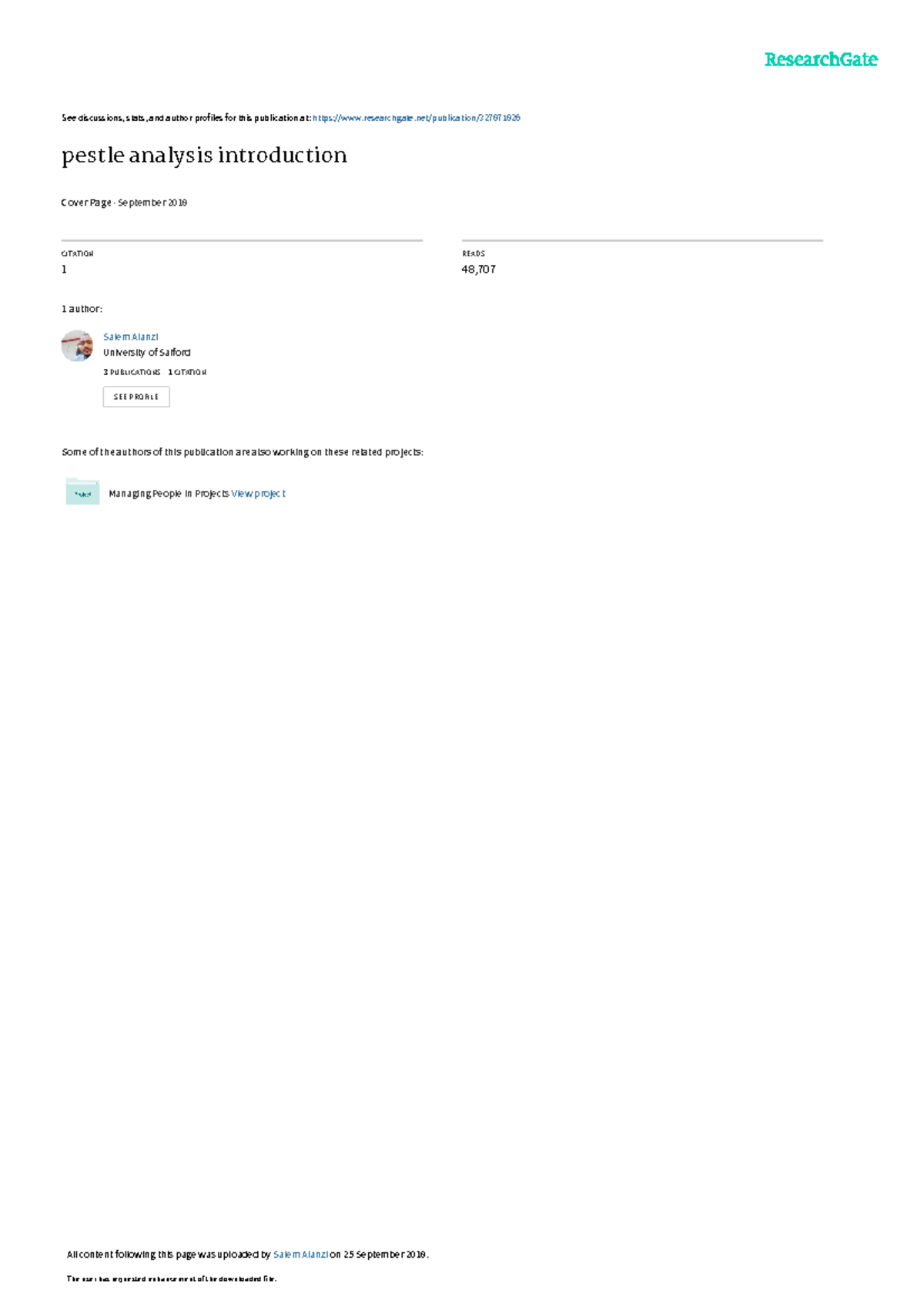The image presents a publication header from ResearchGate, a platform for academic publications. At the top, there's a prompt to "See discussions, stats, and author profiles for this publication" followed by a URL: [https://www.researchgate.net/publication/327871826](https://www.researchgate.net/publication/327871826), highlighted in blue.

Below this, the title "PESTLE Analysis Introduction" appears in plain black font, directly followed by "Cover Page" rendered in bold black text. Next, in smaller, unbolded font, there's a date: "September 2018," though it's hard to read due to low image quality. A light gray divider separates these elements from the rest.

Under the divider, a bolded caption "AUTHOR" appears in black, followed by a photo of a man in the right corner with the name "Salem Alonzi" highlighted in blue. Below his name, it notes "University of Salford" in smaller, gray or black print.

Further down, there's a section titled "PUBLICATIONS" in all caps and bold black font. It lists "three publications," alongside "one citation" in gray capital letters. A light gray-bordered white rectangular icon with "SEE PROFILE" in capital black letters follows.

At the bottom of the image, a bolded black font reads "Some of the authors of this publication are also working on these related projects:" followed by a light blue stretched-out folder icon. The text "Managing People in Projects" appears in blue, and a clickable "View Projects" link in blue completes the layout.

The overall visual is structured with various elements highlighting author information, related projects, and publication details, all set against a professional academic backdrop.